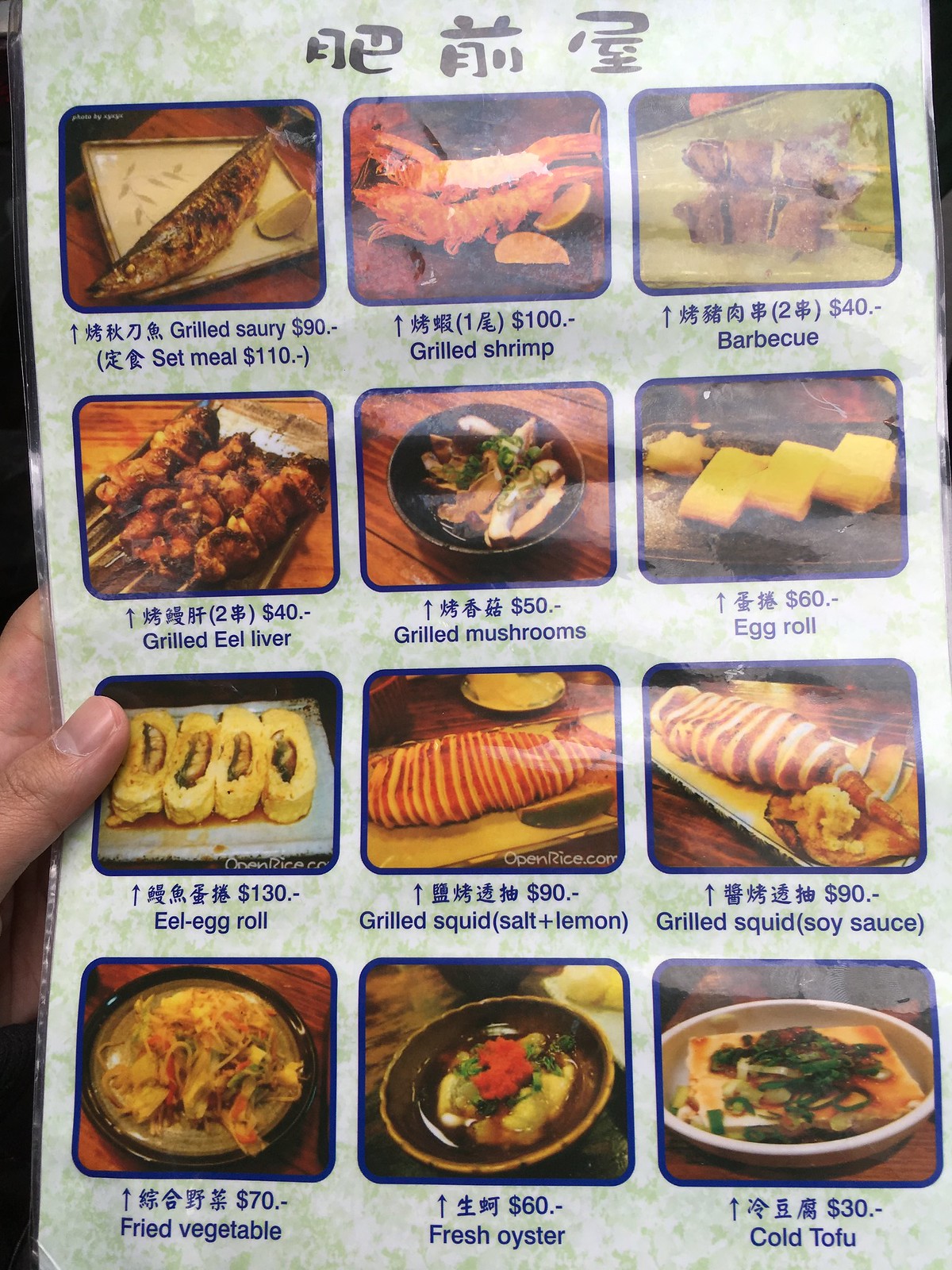In this vibrant color photograph, a neatly manicured hand with light-colored skin can be seen holding a restaurant menu, which appears to be from a Japanese-Chinese fusion eatery. The menu, measuring approximately 18 to 20 inches in height and 11 to 12 inches in width, is laid out in an organized manner, displaying four rows of menu items. Each row contains three sections accompanied by vivid color photographs of the dishes, their names, and prices. The selection showcases traditional Asian cuisine, featuring dishes such as egg rolls, grilled fish, and fried vegetables. The hand gripping the menu provides a sense of scale and human element to the image, hinting at the attentive and inviting atmosphere of the restaurant.